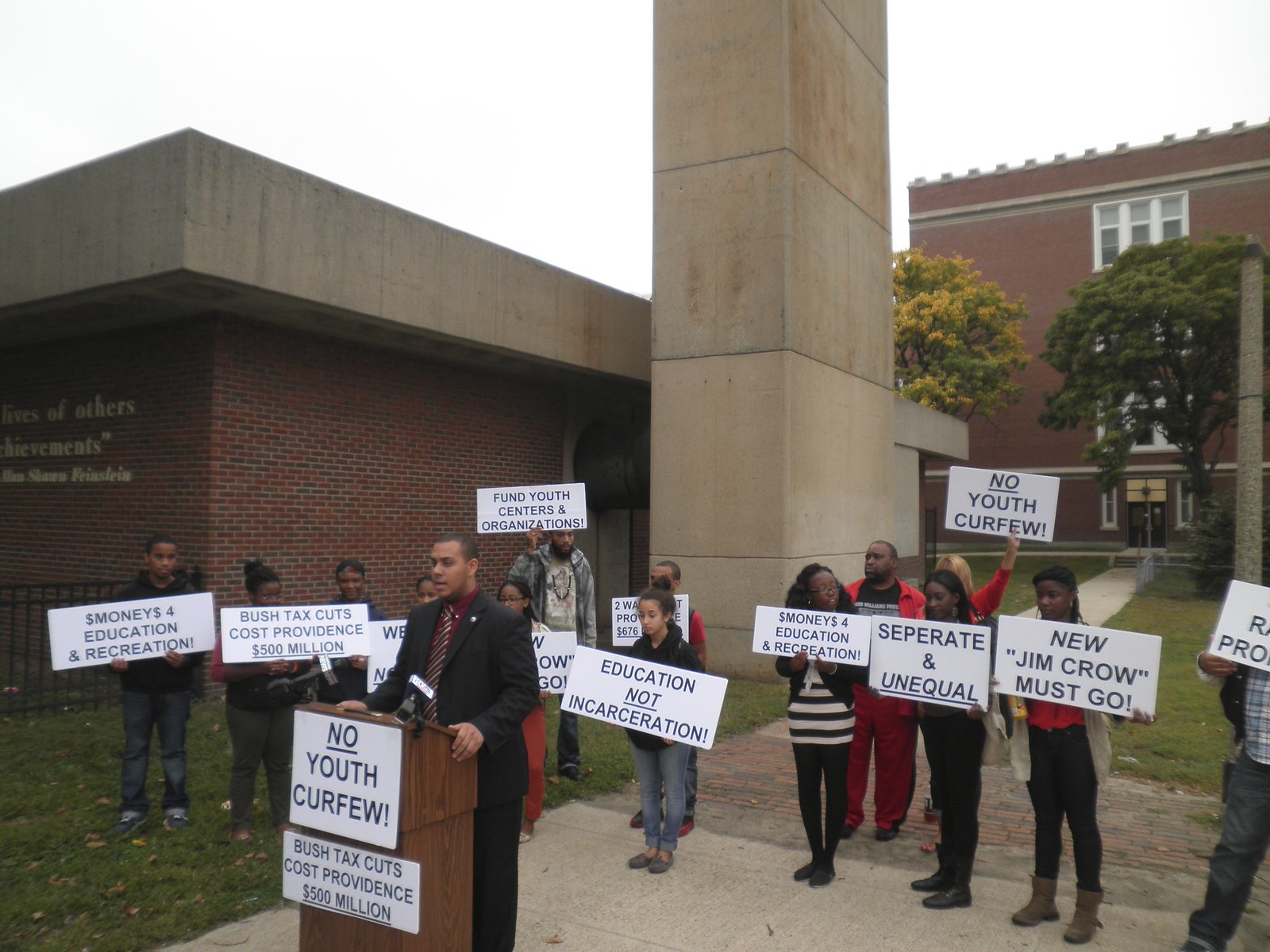This image captures a dynamic protest scene outside a red brick building, which resembles a school. Predominantly featuring African American individuals, the photo centers on a black man standing behind a wooden podium equipped with a microphone. In front of the podium, a sign reads "No Youth Curfew" and "Bush Tax Cuts Cost Providence $500 Million." The protesters surrounding him hold various white signs with blue lettering, advocating for “Money for Education and Recreation," "Education Not Incarceration," "Separate and Unequal," and "New Jim Crow Must Go." The background reveals more of the red brick structure with distinctive large concrete blocks and a substantial roofline. Trees frame the scene, leading up to a doorway, enhancing the setting’s civic and communal atmosphere. The protester's visible passion underscores the collective demand for equitable education and opposition to youth curfews and economic policies perceived as detrimental to the community.